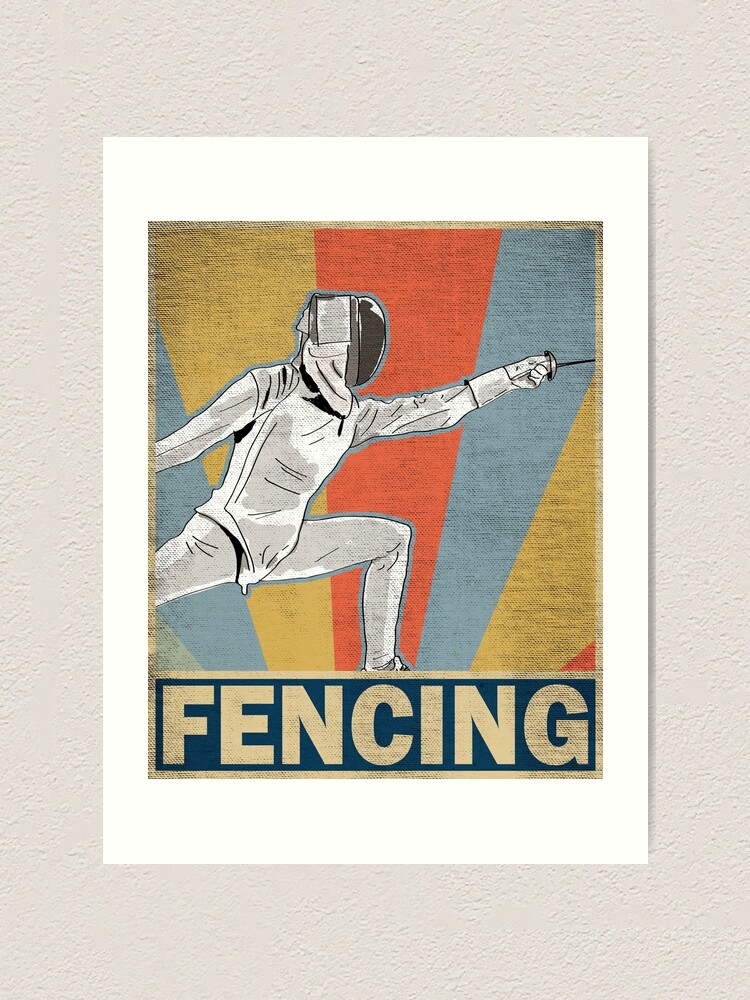This is a photograph of a poster hanging on a white, textured wall. The poster, designed with a grungy, rustic aesthetic reminiscent of Shepard Fairey's style, centers on the dynamic image of a fencer in full uniform. The fencer, captured in a deep lunge with a saber extended, has a reflective helmet and is set against a vibrant backdrop of segmented, colorful rays in teal, blue, yellow, and orange. The rays fan out dramatically in the classic "Hope" poster style, giving the scene an energetic, vintage feel. The word "FENCING" is boldly displayed in tan caps below the fencer's outstretched left foot, with their right arm extending beyond the left border of the image, emphasizing motion and action. The whole scene is encapsulated within a digital art template with a white border, tailored for inserting custom artwork.